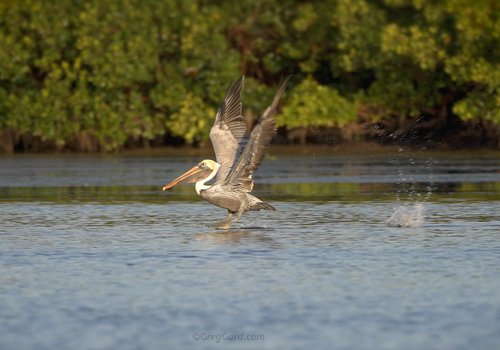In this vibrant, landscape-oriented color photograph, a pelican is dramatically captured in the center of the frame as it appears to either land or take off from the dark greenish-blue surface of a body of water. The pelican is in profile, facing the left side, with its wings impressively outstretched above its head. Its long yellow beak contrasts sharply with its white head and curved neck, while its body is a mix of light gray and light brown feathers, with darker shades accentuating the wing tips. Just behind its skimming feet, a splash disrupts the water's surface, suggesting recent movement or a possible catch.

The lower half of the image is dominated by the water, vibrant with hues of green and blue, while the upper half showcases a lush backdrop of dense green trees and plants. These trees extend from the top left to the top right, framing the scene with their rich, leafy presence. The image, marked by its photographic realism, is devoid of any text, allowing the natural beauty and dynamic motion to take center stage, highlighting the pelican's interaction with its aquatic environment.